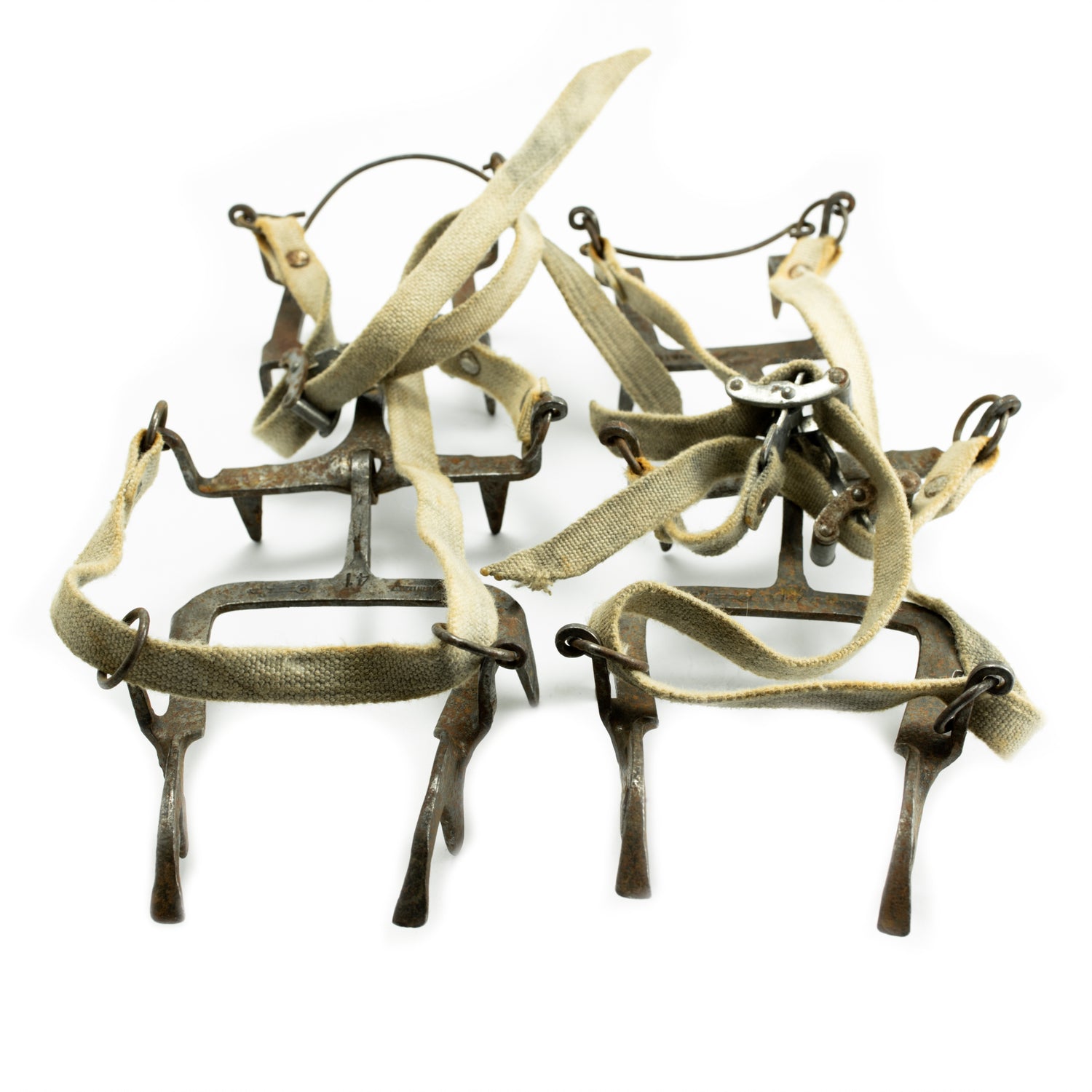The image depicts a pair of old metal crampons set against a plain white background. The crampons, designed to be attached to shoes to provide better traction on ice, feature spiked metal plates with rusty patches indicative of their age. They are connected by a hinge with a hook mechanism that allows one piece to latch into the other. The crampons are secured with discolored white laces, now showing yellowing edges, threaded through metal rings and additional metal holdings. These structures allow the laces to be looped and locked, ensuring the crampons stay firmly in place when used. The simplicity of the white background highlights the intricate details and aged characteristics of these metal contraptions.